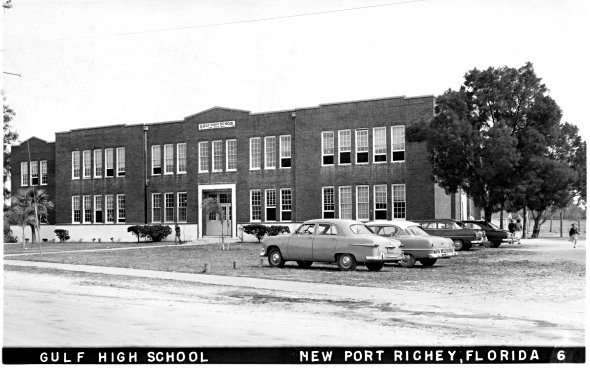This black-and-white photograph, likely taken in the 1960s or 70s, captures the exterior of Gulf High School, located in Newport Ritchie, Florida. At the very bottom of the image, a black bar with capitalized white font reads "Gulf High School, Newport Ritchie, Florida 6." The school building, constructed from a darker-colored brick or stone, spans two stories and features numerous long rectangular windows, some of which are open. In front of the school, four vintage cars, likely from the 1950s or 60s, are parked on what appears to be a worn grass area rather than a traditional paved lot. Several trees, including large ones to the right and various smaller bushes and palm trees near the entrance, add to the school's landscape. A few students, dressed in dark tops and light bottoms resembling uniforms, can be seen scattered around, with one notably walking away from the camera. A partially visible road runs to the left of the parking area, enhancing the scene of an active school day.